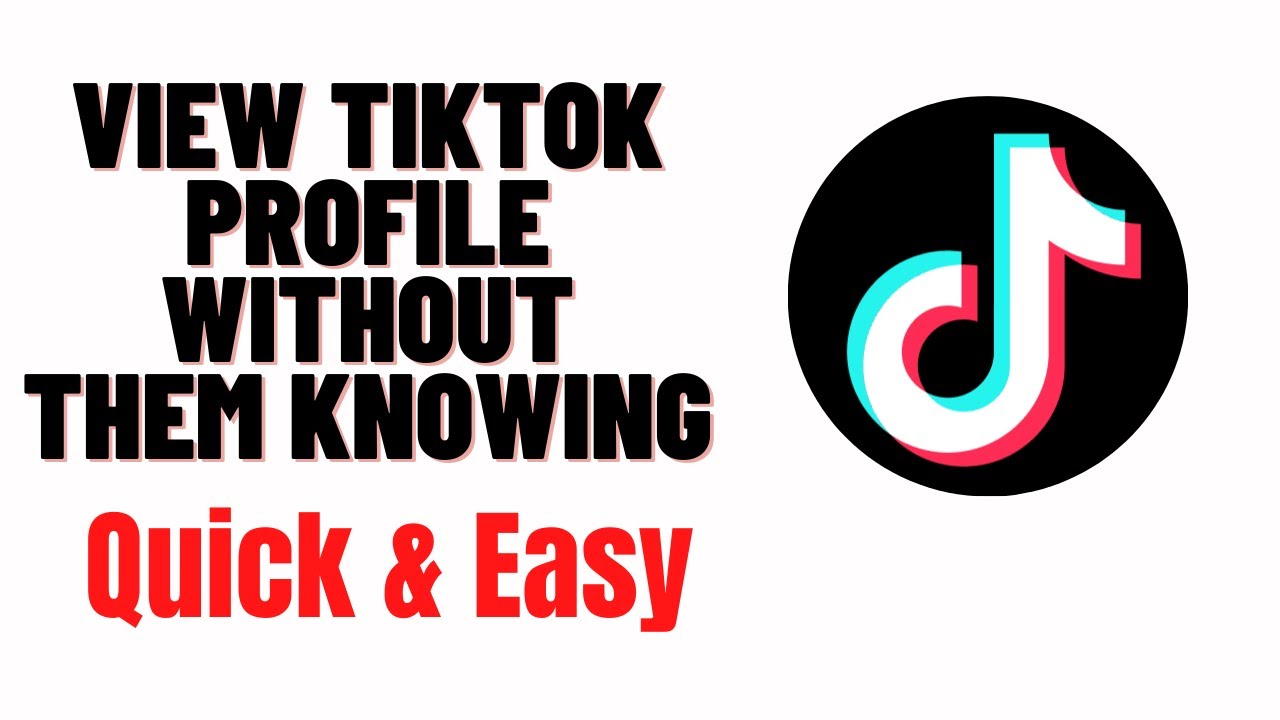The image features a large caption on the left side that reads, "View TikTok profile without them knowing. Quick and easy." The majority of the text is in black, except for "Quick and easy," which is highlighted in red. On the right side of the image, there is the TikTok logo, represented by a black circle containing a stylized, multicolored symbol resembling a lowercase 'd' in white, baby blue, and dark pink. The background color of the image is entirely white, providing a stark contrast to both the text and the logo, making them stand out prominently.